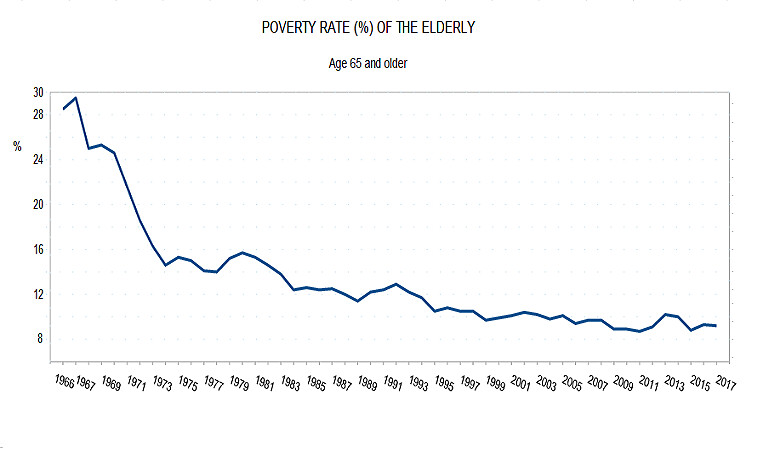The image displays a detailed line chart titled "Poverty Rate of the Elderly (Ages 65 and Older)," tracking changes in the percentage of elderly individuals in poverty over time. The x-axis spans from 1966 to 2017 in two-year increments, while the y-axis ranges from 8% to 30% in four percent increments. The primary visual feature is a dark blue line indicating the poverty rate over the years. Starting at about 28% in 1966, the line shows a sharp decline to around 15% by 1973. Following this, the rate remains relatively stable with minor fluctuations: a small increase, then a decrease, and slight rises between 1989 and 1995. A plateau persists up till approximately 2011, after which there's an upward trend, concluding near 10% in 2017. Although the chart does not specify the country, it is presumed to represent the United States based on its English annotations. The graphical presentation is predominantly monochrome except for the blue line illustrating the data.